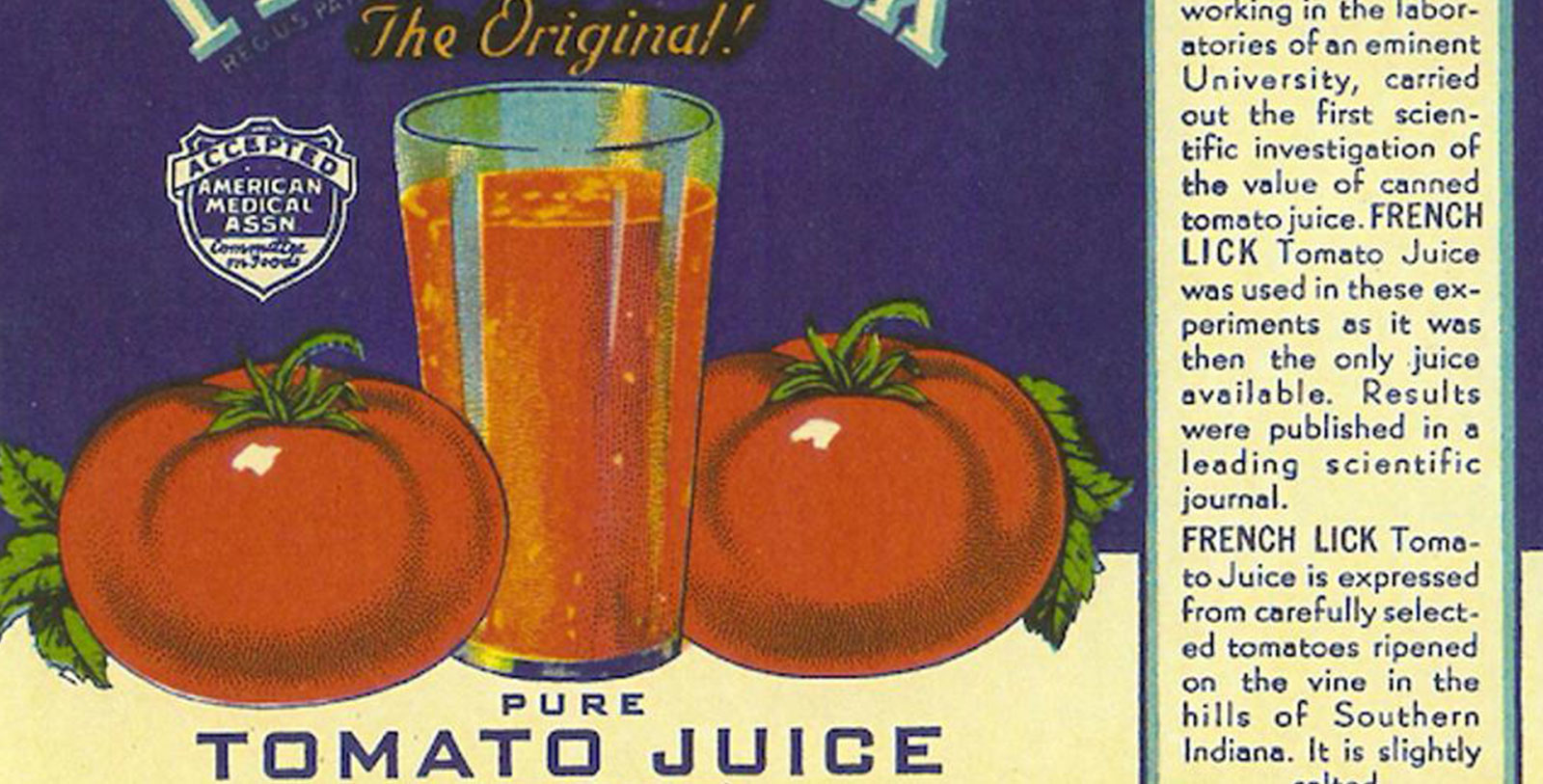The label featured in this image provides comprehensive information about a canned tomato juice product. On the right side, there is an illustration that outlines the ingredients used in the juice. The label itself is predominantly light brown with blue accents. An accompanying blueprint highlights a scientific investigation into the nutritional value of canned tomato juice, specifically noting that French-Licked Tomato Juice was utilized in these experiments due to its availability at the time.

The main section of the label prominently displays a blue background with "French-Licked" written in bold white letters and "original" highlighted in yellow. Additionally, it features the "Accepted" tag from the American Medical Association, signifying its endorsement. Central to the design is an image of a large glass filled with tomato juice, flanked by two large, ripe tomatoes on either side. The phrase "pure tomato juice" is clearly written in blue, emphasizing the product's quality and purity.